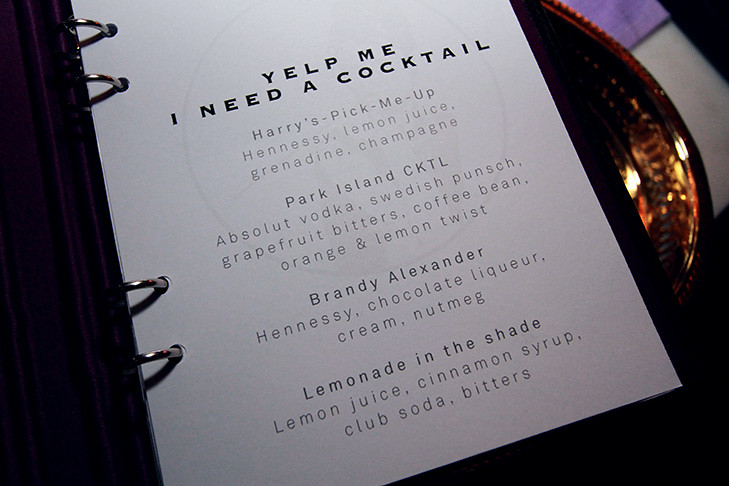The image depicts a detailed menu page from a spiral-bound binder, adorned with four metal rings on the left side. The page rests against a shiny gold dinnerware piece, visible in the upper right corner. The top of the page features the bold black text, "Yelp me, I need a cocktail." Below, there is a list of cocktails accompanied by their ingredients in lighter gray text. The cocktails include:

1. **Harry's Pick-Me-Up:** Hennessy, lemon juice, grenadine, champagne.
2. **Park Island CKTL:** Absolut Vodka, Swedish Punch, grapefruit bitters, coffee bean, orange, and lemon twist.
3. **Brandy Alexander:** Hennessy, chocolate liqueur, cream, nutmeg.
4. **Lemonade in the Shade:** Lemon juice, cinnamon syrup, club soda, bitters.

The page also features a light gray circle design in the background, enhancing the menu's aesthetic.